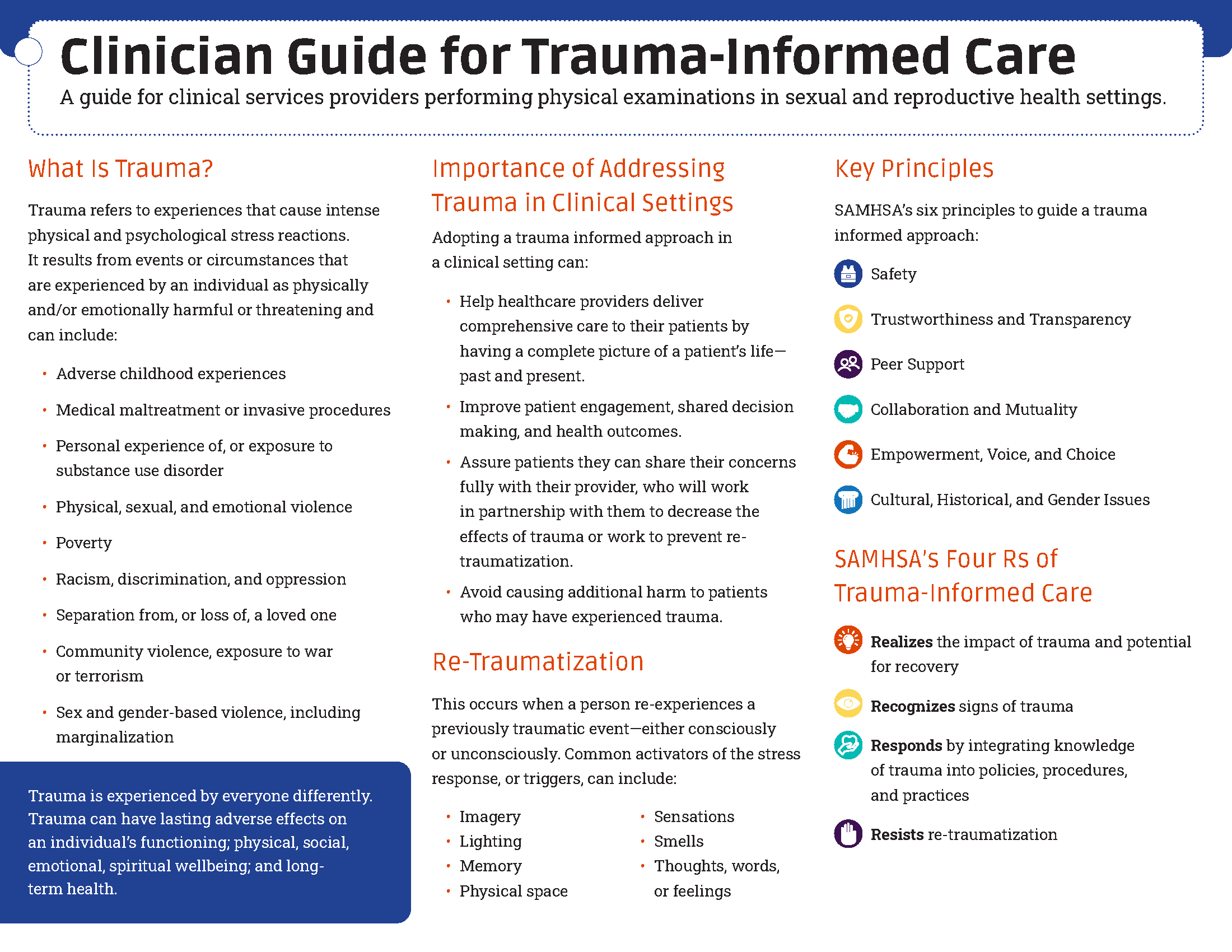The image is a detailed page from a textbook or pamphlet titled "Clinician Guide for Trauma-Informed Care: A Guide for Clinical Services Providers Performing Physical Examinations in Sexual and Reproductive Health Settings." It is a landscape-oriented page, wider than it is tall, with a predominantly white background and black text. There is a thin blue border at the top and a more pronounced dark blue inset in the bottom left corner. The inset reads, "Trauma is experienced by everyone differently. Trauma can have lasting adverse effects on an individual's functioning, physical, social, emotional, spiritual well-being, and long-term health."

The guide is organized into several sections with title headings in an orange-red font. These sections are: "What is Trauma," "Importance of Addressing Trauma in Clinical Settings," "Re-traumatization," "Key Principles," and "SAMHSA's Four R's of Trauma-Informed Care." Each of these sections contains additional black text providing detailed descriptions and bullet points. 

Specifically, the "Key Principles" section lists SAMHSA's six principles to guide a trauma-informed approach, which include: Safety, Trustworthiness and Transparency, Peer Support, Collaboration and Mutuality, Empowerment, Voice and Choice, and Cultural, Historical, and Gender Issues. The "SAMHSA's Four R's of Trauma-Informed Care" section outlines essential practices: realizing the impact of trauma and the potential for recovery, recognizing signs of trauma, responding by integrating knowledge of trauma into policies, procedures, and practices, and resisting re-traumatization. Colorful icons accompany the explanations of these principles and the "Four R's," enhancing the guide's visual appeal.